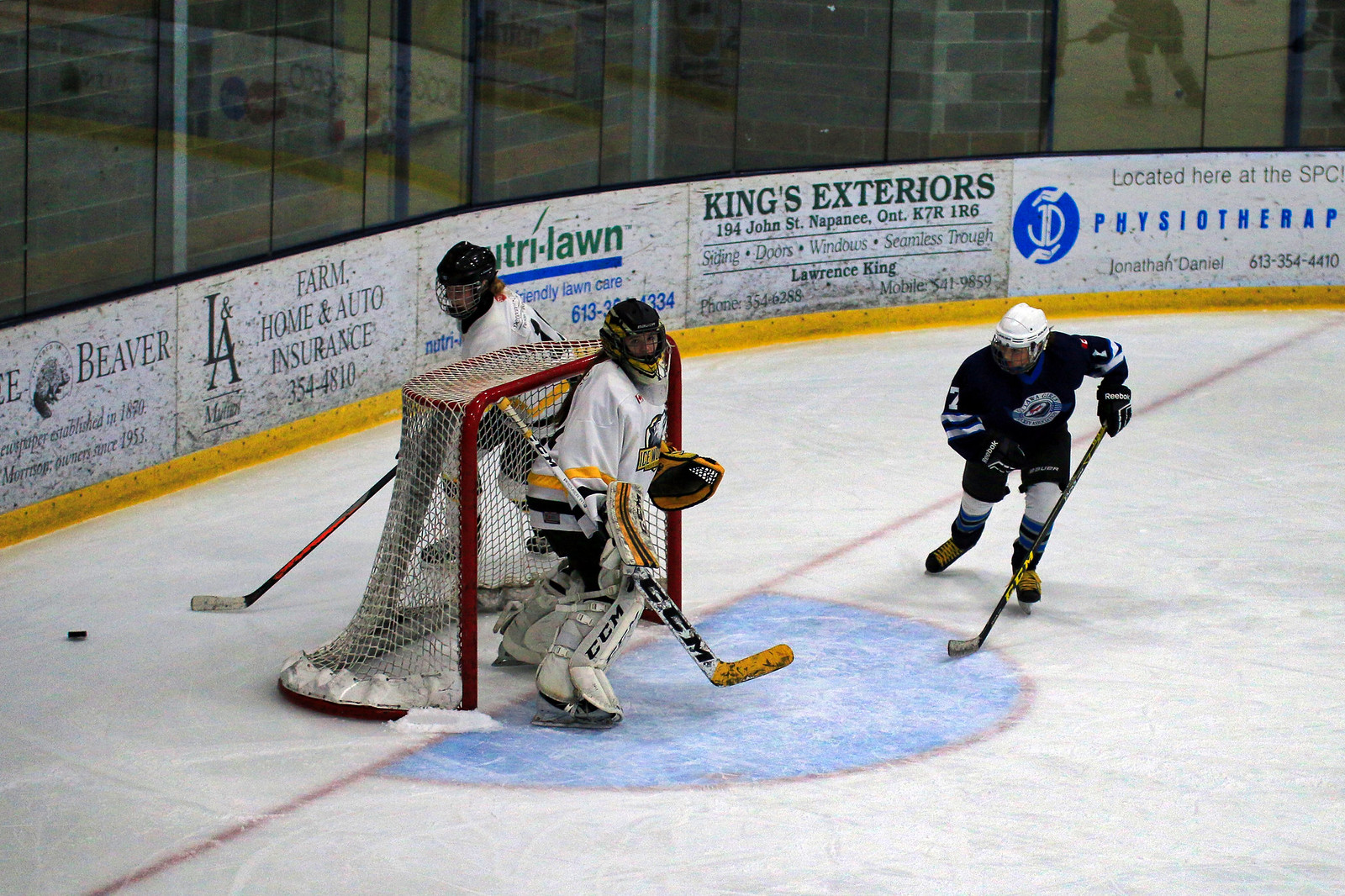In this horizontally aligned rectangular picture, three players are actively involved in an ice hockey game. The ice, a mix of white and gray with visible scrapes, showcases the intensity of the match. In front of the worn, small-netted goal, a goalie stands poised, adorned in white gear with yellow and black stripes. His equipment includes a noticeably yellow stick and a black glove, and his skate prominently features the branding "CCM."

Just outside the goalie's area, a player in a black jersey and shorts, paired with a white helmet and yellow skates, is in position. Another player from the opposing team, distinguishable by his white jersey, is focused on securing the puck to the left of the scene.

The backdrop includes a short wall separating the rink from the stands, which bears a rugged appearance and is adorned with sponsors' advertisements such as King's Exteriors, Physiotherapy, and Farm Home and Auto Insurance. Above this wall, tall windows allow additional light into the lively, competitive atmosphere of the rink.